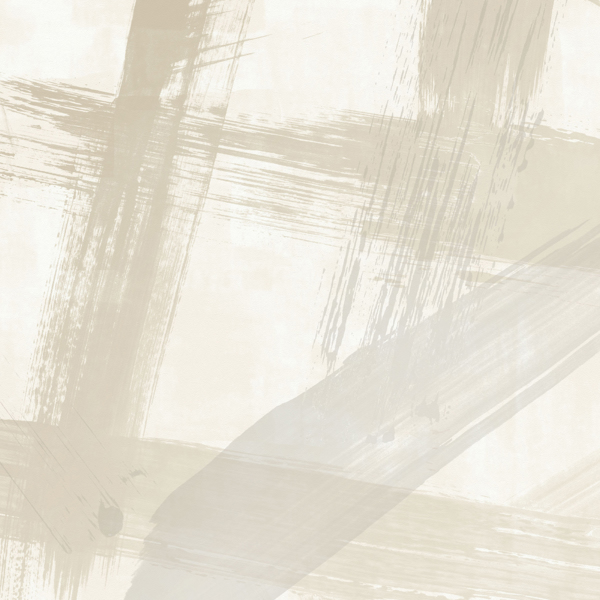This image depicts a modern abstract painting that is nearly square in dimension. The background is a pale beige hue, which gives an almost off-white or very light gray appearance. The painting is characterized by a series of brush strokes that traverse the canvas in various directions, creating an intricate pattern of lines. These strokes are neither too thin nor too thick, occupying a moderate width, and consist of shades ranging from a darker beige to different tones of gray, including light gray and summit gray. The lines are primarily straight, with some featuring subtle curves, adding to the abstract nature of the artwork. The composition lacks any bold colors, signatures, or watermarks, focusing solely on the nuanced interplay of beige and gray brush strokes against the subdued background.